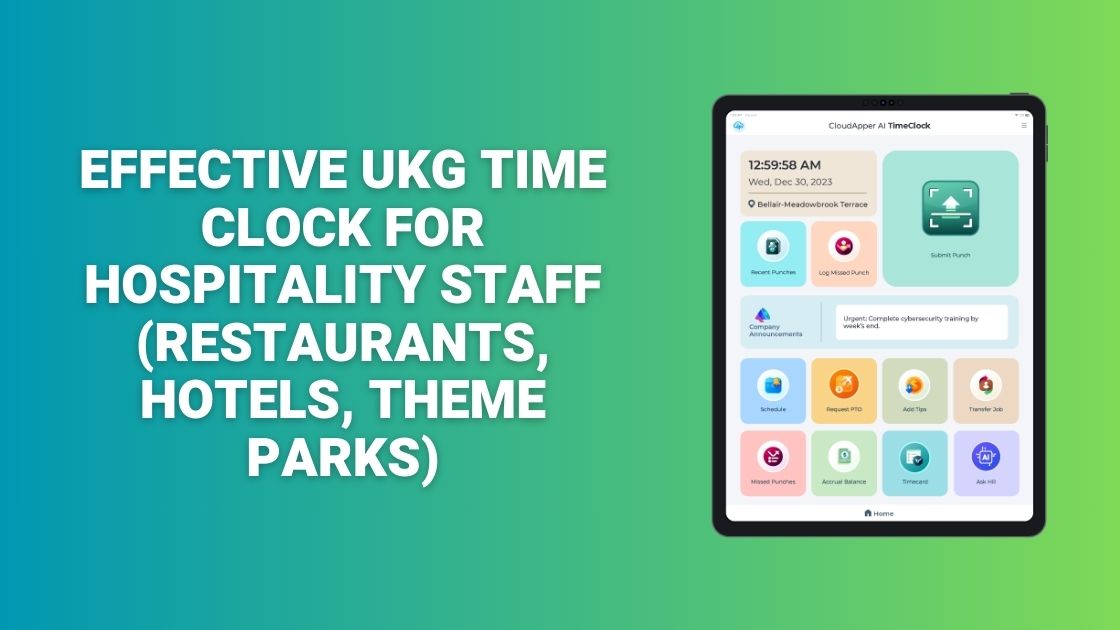This horizontal, landscape-oriented advertisement, approximately one and a half times wider than it is tall, features a gradient background transitioning from teal on the left to a bright lime green on the right. On the left-hand side, centered text in white, all capital letters, reads: "EFFECTIVE UKG TIME CLOCK FOR HOSPITALITY STAFF, RESTAURANTS, HOTELS, THEME PARKS". To the right, an image of a tablet or iPad displays a control panel interface. The screen on the tablet features several navigation tiles: the top half includes two big squares, with the left one subdivided into three smaller parts. Below this, a rectangle spans the width of the screen, followed by eight color-coded squares at the bottom, each with different symbols, presumably representing various functions of the app. This detailed assembly suggests that the depicted app is likely for managing schedules or other functions relevant to hospitality staff.